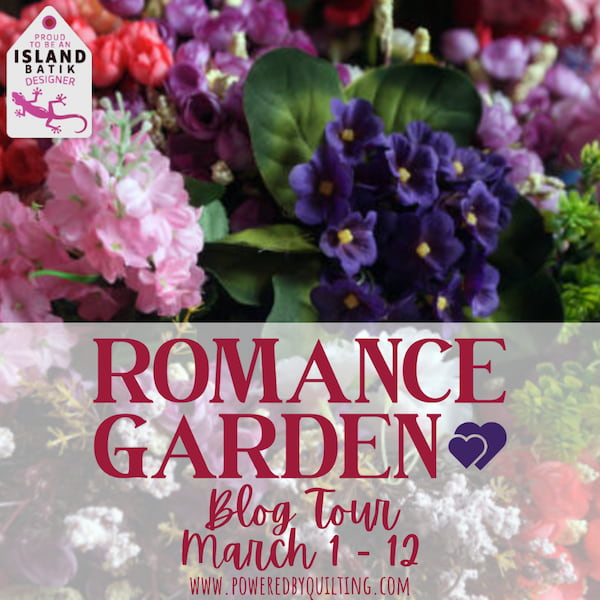The image is an advertisement for a blog tour, prominently featuring a vivid photograph of various flowers and greenery. In the background, an arrangement of flowers includes shades of pink, orange, dark pink, and purple, complemented by a few green leaves, some appearing slightly artificial with visible strings. Overlaying this botanical display is a semi-transparent, white-tinted rectangle at the bottom, allowing the vibrant florals to show through while housing key text details. The text within this rectangle reads: “Romance Garden,” adorned with two small purple hearts on either side of the word “Garden.” Below this, it announces a “blog tour, March 1st through the 12th” and provides the URL: “www.poweredbyquilting.com.”

In the top left corner, a distinctive label declares, “Proud to be an Island Batik Designer,” next to the silhouette of a pink gecko lizard, subtly hinting at an island or tropical theme. This detailed and colorful composition effectively highlights the nature of the event and its association with quilting, making it a captivating and informative visual advertisement.